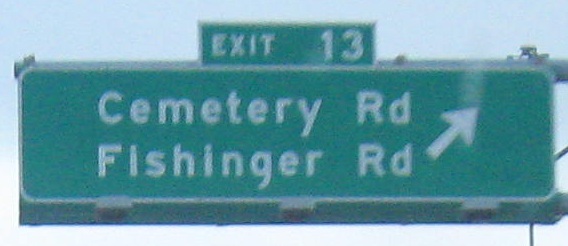The rectangular image captures a prominent street sign against a backdrop of a clear, light blue sky. Dominating the frame from left to right and top to bottom, the green street sign features a thin white border and houses the name "Cemetery Rd," with "RD" being the abbreviation for road, written in bold white lettering. Directly below "Cemetery Rd," the sign displays "Fishinger Rd" along with a diagonal white arrow pointing towards the upper right-hand corner, indicating the direction to Fishinger Road. Above this portion of the sign, a smaller green rectangle presents the word "Exit" alongside the number "13" in white, providing additional navigational information. The high contrast between the green signage and the crisp blue sky makes the details easily readable and visually striking.